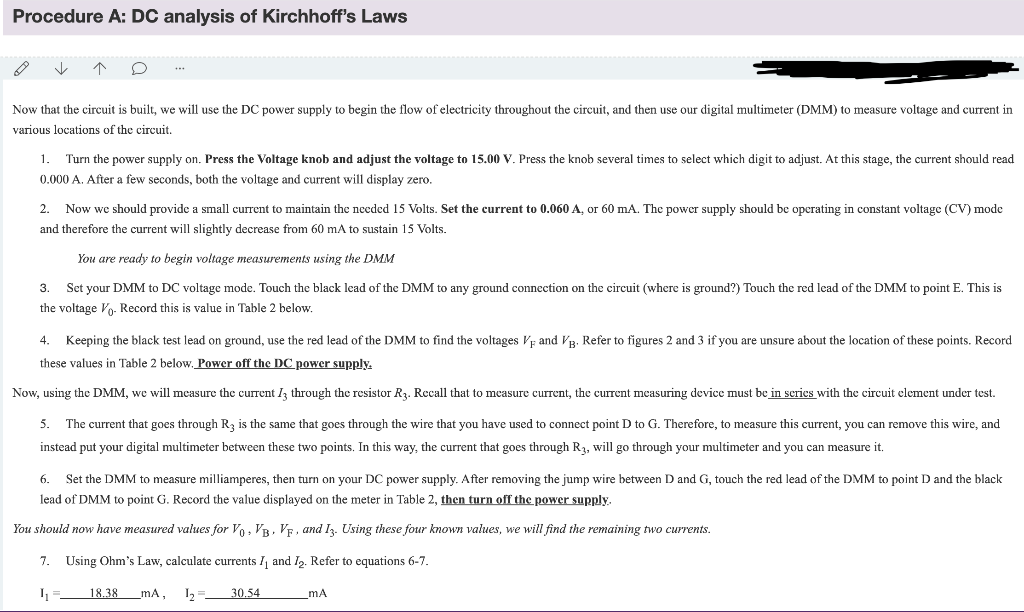This horizontal rectangular image presents a detailed procedural guide for conducting an analysis of Kirchhoff's Laws in DC circuits. The top section of the image features a light gray banner running horizontally from left to right, displaying bold black text which reads: "Procedure A: DC Analysis of Kirchhoff's Laws."

In the main body of the image, there is a white horizontal strip followed by a light blue section containing some icons on the left side and some text crossed out with black Sharpie on the right. Under this, in a white area, the following instructions are presented in black font:

1. "Now that the circuit is built, we will use the DC power supply to begin the flow of electricity throughout the circuit. Then use our digital multimeter (DMM) to measure voltage and current in various locations of the circuit."

Indented, the steps continue:

1. Turn the power supply on. In bold font, "Press the voltage knob and adjust the voltage to 15.00V." Non-bold font instructions note, "Press the knob several times to select which digit to adjust. At this stage, the current should read 0.000A. After a few seconds, both the voltage and current will display zero."

2. Now we should provide a small current to maintain the needed 15 volts. In bold font, "Set the current to 0.060A," followed by non-bold text, "or 60mA. The power supply should be operating in constant voltage (CV) mode, and therefore the current will slightly decrease from 60mA to sustain 15 volts. You are ready to begin voltage measurement using the DMM."

3. "Set your DMM to DC voltage mode. Connect the black lead of the DMM to any ground connection on the circuit (where is ground?). Touch the red lead of the DMM to point E (denoted as V₀). Record this value in table two shown below."

4. "Keeping the black lead on ground, use the red lead of the DMM to find the voltages V_F and V_B. Refer to figures two and three if you are unsure about the location of these points. Record these values in table two below." In bold and underlined, "Power off the DC power supply."

Non-bold text continues: "Now using the DMM, we will measure the current I through the resistor R₃. Recall that to measure current, the current measuring device must be in series with the current element under test."

5. "The current that goes through R₃ is the same that goes through the wire connecting point D to G. Therefore, to measure the current, you can remove the wire and instead put your digital multimeter between these two points. This way, the current that goes through R₃ will go through your multimeter, and you can measure it."

6. "Set the DMM to measure milliamperes, then turn on your DC power supply. After removing the jump wire between D and G, touch the red lead of the DMM to point D and the black lead of the DMM to point G. Record the value displayed on the meter in table two." In bold and underlined, "Then turn off the power supply."

Non-bold text further states: "You should now have measured values for V₀, V_B, V_F, and I₃. Using these four known values, we will find the remaining two currents."

7. "Using Ohm's law, calculate currents I₁ and I₂. Refer to equations six to seven."

The image concludes with a small formula, finalizing the detailed procedural guide.